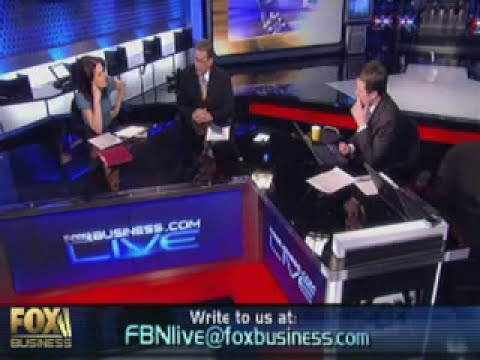The image shows an indoor scene of a newsroom featuring three newscasters—two men and one woman—engaged in conversation at an L-shaped news desk. The woman is positioned on the left side of the desk, and she appears to be speaking to the two men: one seated to her immediate right and the other across from her. The desk displays the words "live" in blue letters on both the left and right sides. The bottom left-hand corner of the image prominently features the text "Fox Business" in gold letters, while the center bottom of the image shows the contact information "write to us at fbnlive@foxbusiness.com" in blue letters. The backdrop includes a blue wall in the upper left corner, and the floor appears to be white and black. On the desk, there is a yellow coffee cup, several sheets of paper, a binder, and two notes. The background behind the anchors includes a long desk with a laptop and what might be a landline phone, suggesting a typical newsroom environment. The overall scene appears to be a screenshot of a newscast, though it is somewhat pixelated, indicating poor image quality.